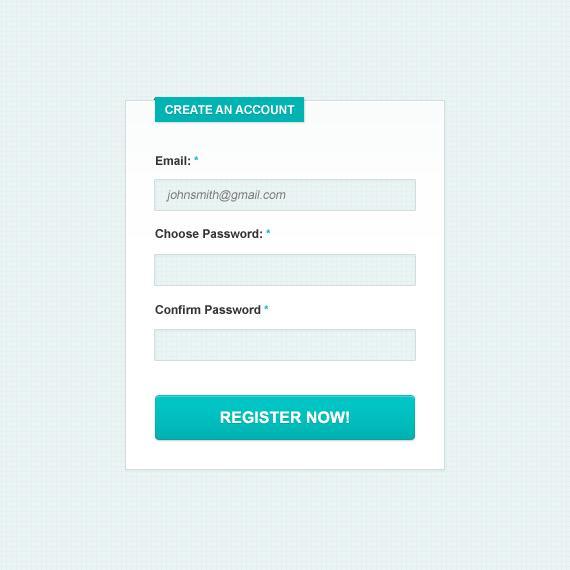A screen capture of a website's registration page is depicted. The page features a very pale mint green background, with a prominent white registration box in the center. The registration form includes several key elements, all neatly organized for user convenience. The first dark green button with white text reads "Create an Account." Below this, there is a designated field for email entry, highlighted by an "Email:" label and marked with a green asterisk to indicate a required field. The example email entry "johnsmith@gmail.com" is pre-filled in this field.

Following the email field, there is a "Choose Password:" label, also accompanied by a green asterisk, denoting another required field. This section contains a blank text box for users to input their desired password. Subsequently, the "Confirm Password:" label appears, again marked with a green asterisk. This is followed by another blank text box for password confirmation.

At the bottom of the registration form, there is a second dark green button with white text that enthusiastically instructs users to "Register Now!" This detailed and user-friendly interface outlines everything needed to create an account on the website.